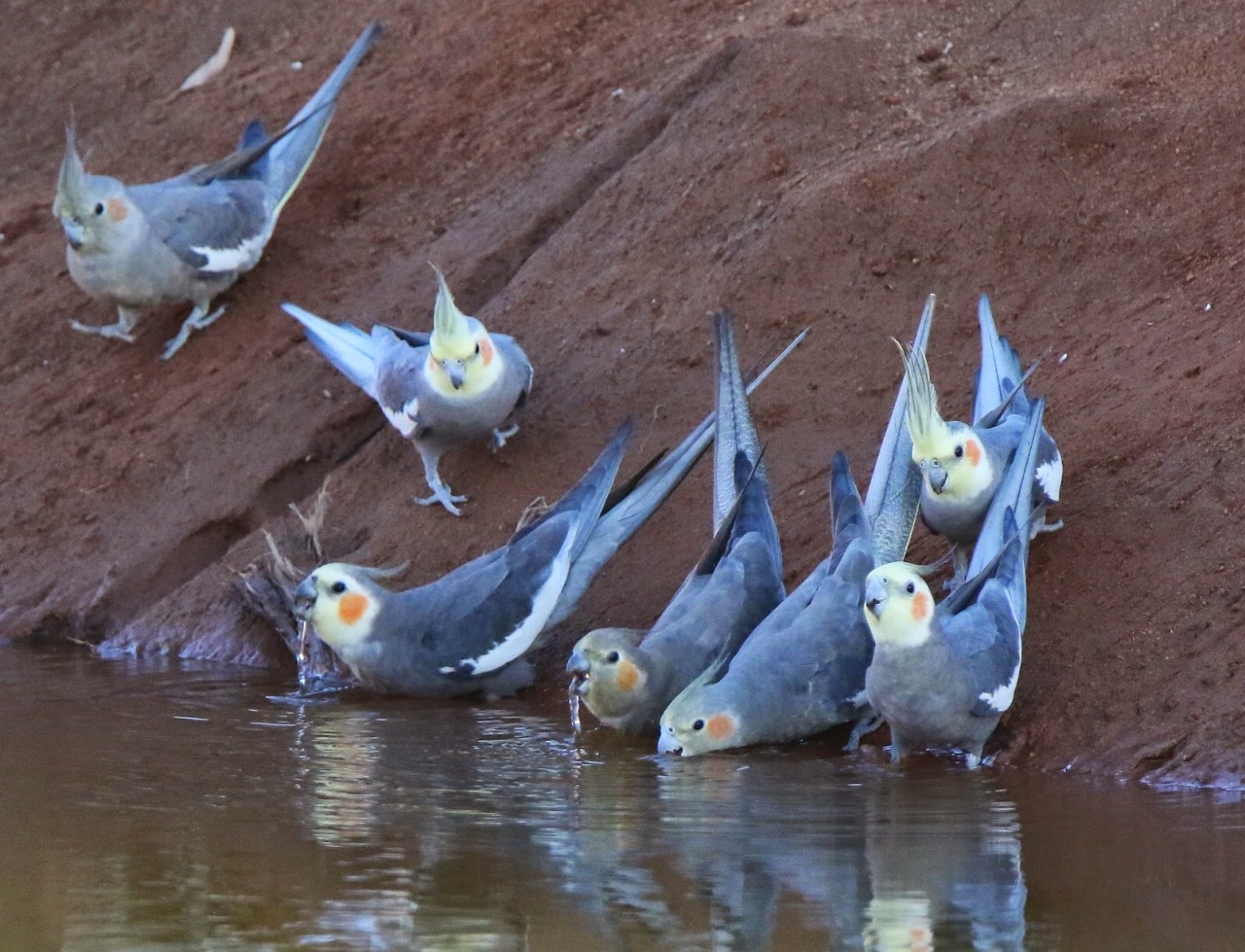The image captures a serene scene of seven cockatiel-like birds gathered at the edge of a murky brown-green creek, surrounded by dark brown and red-brown soil. Five of the birds are positioned almost right at the water's edge, with four of them dipping their beaks into the water to drink. One bird has its beak slightly raised with a droplet of water forming, while another is in the process of lowering its head to take a sip. A sixth bird has one foot tentatively in the water, with a seventh bird close behind it, also preparing to drink. Two birds linger a bit further back from the water. The birds are characterized by their grayish bodies and vibrant heads, adorned with a mix of blue and cream-colored feathers, crowned with crested feathers above their beaks. Their faces feature striking rosy orange cheeks, adding to their vivid appearance. Off to the top left corner of the image, a loose feather can be seen, contributing to the natural, untouched feel of the setting. The overall scene depicts a quiet moment in the wild, accentuated by the birds' colorful plumage against the earthy tones of the creek bank.